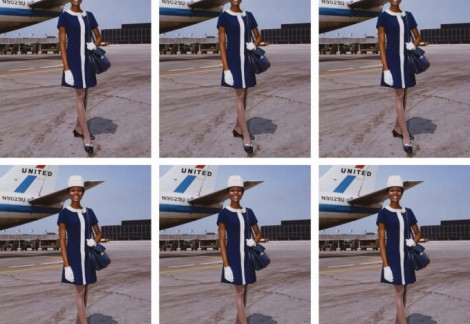The collage features six photos arranged in two rows and three columns, capturing various angles of an African American flight attendant from the 1970s or 1980s. She is smiling and dressed in a stylish dark blue mini dress with white trim around the neckline and a white stripe running down the front. She accessorizes with white gloves, a white hat, and black pointed shoes. She also carries a blue carry-on bag slung over her left shoulder. In the top three photos, her head is cropped out, showing her from the neck down to her shoes, standing on the runway with a United Airlines plane in the backdrop. In the bottom three photos, her feet are cropped out, providing a clear view of her face and hat, with more visible details of the white plane bearing the United logo, and red and blue stripes in the background. The photos appear to be taken on an airport tarmac as she poses gracefully in front of the airliner.